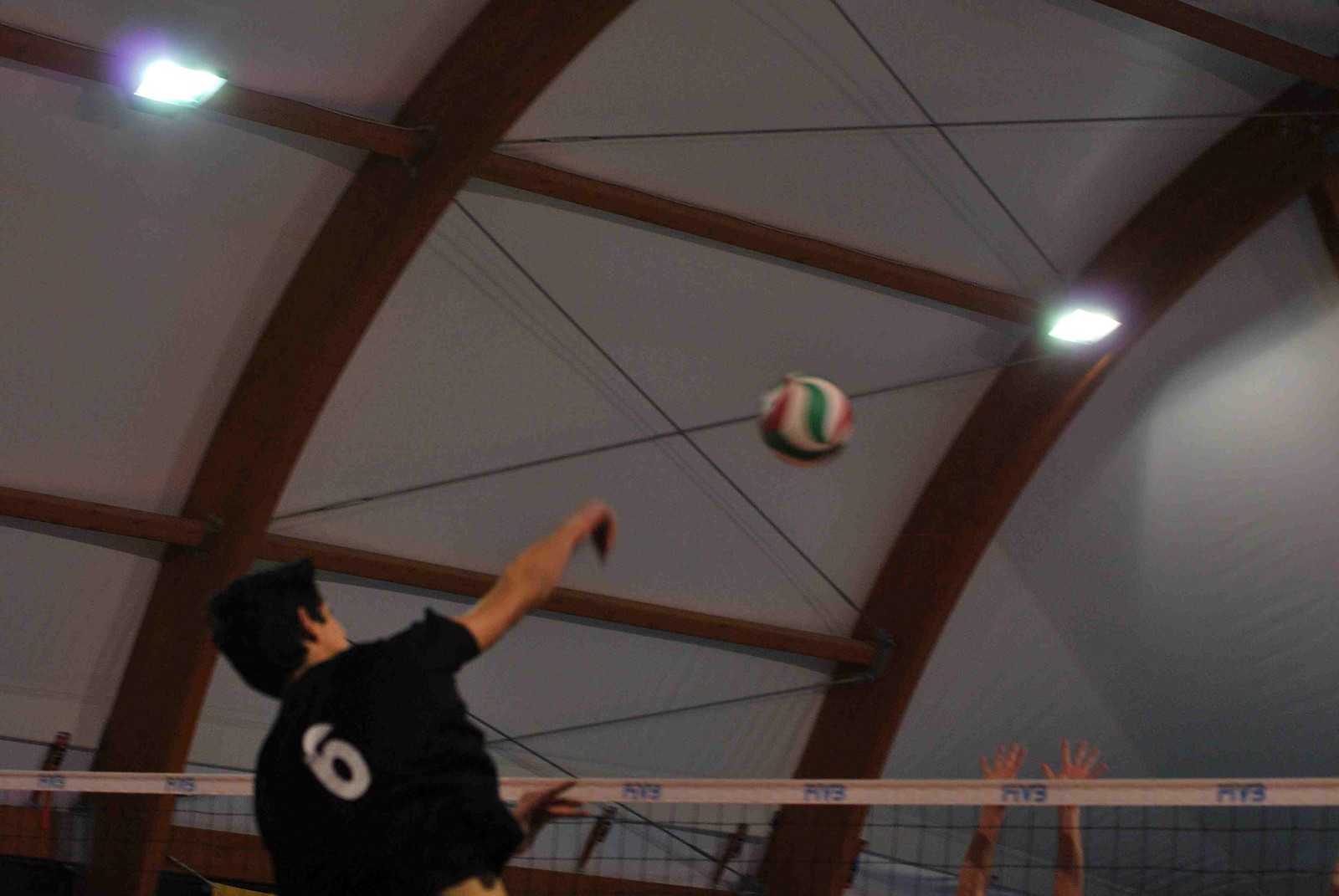The photograph captures an intense moment inside a unique sporting complex with a distinctive arched wooden ceiling made of thick beams interlaced with wires. The building's architecture gives it a dome-like appearance, reminiscent of a large tent. The scene focuses on a volleyball match, highlighting a player in mid-action. Wearing a black short-sleeved jersey with the number six in white, the player, who has short black hair and light skin, appears to have just launched the red, white, and green swirl-patterned volleyball over the net. The action shot shows his right arm raised and hand pointed downwards as the ball blurs in motion. He has gained significant height, leaping head and shoulders above the net. On the opposing side, two hands reach up, ready to counter the incoming ball. Bright ceiling lights illuminate the indoor venue, adding to the dynamic energy of the moment. The photo, bordered in white with the letters RV3 at the top, perfectly captures the thrilling essence of competitive volleyball.